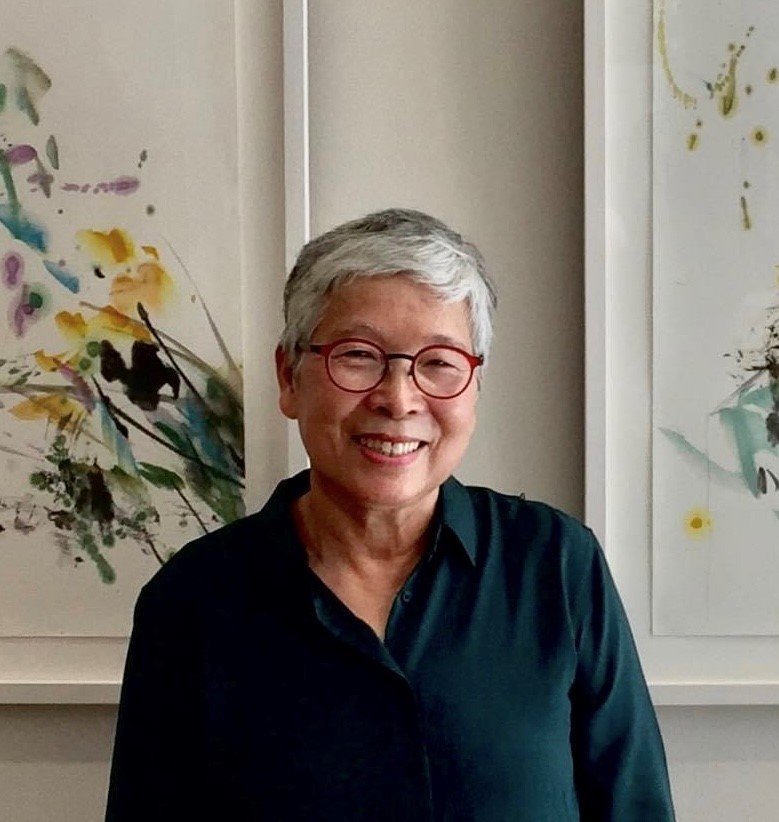The photograph captures an elderly Asian woman, appearing to be in her late 50s or early 60s. She has short white and dark gray hair, and she is smiling warmly, revealing her upper teeth. She is dressed in a long-sleeved, green collared shirt with a three-button polo-style neckline, all buttons left unbuttoned. Her vivid red, round glasses frame her face, adding a touch of vibrancy. The background reveals she is indoors, standing slightly left of center against a beige-colored wall. Behind her are two large, partially visible abstract watercolor paintings. These artworks feature splotches of purples, blues, yellows, blacks, and greens, evoking an impression of wildflowers in a vivid yet abstract style.